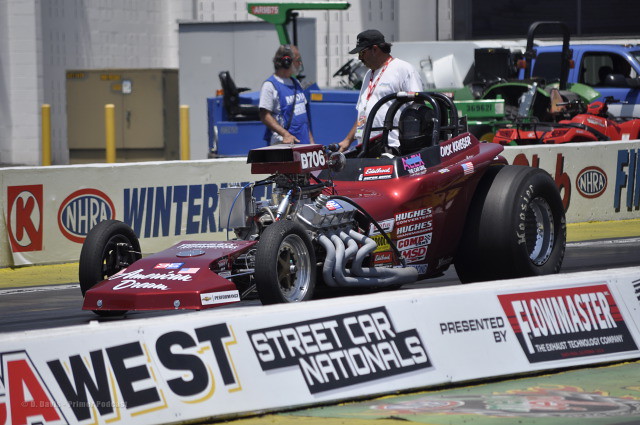The image showcases a vibrant racing scene at the Streetcar Nationals, presented by Flowmaster and NHRA. Prominently featured is a red race car, marked with the number B706, adorned with various sponsor stickers including COMP, MSD, and several others. The powerful engine is strikingly visible with a black roll cage encasing it. Inside the car, the driver is equipped with a black helmet. The race car's design includes significantly larger rear wheels compared to the front, enhancing its streamlined, aggressive look.

In the background, the racetrack is flanked by banners displaying sponsorships and logos. Among the activity, two individuals, likely part of the pit crew, are engaged in conversation; one wears a black baseball cap, has dark hair, a white shirt, and a red lanyard, while the other sports a blue vest with white lettering over a white t-shirt and has light curly hair. Additional elements in the background include other race cars, a dumpster, and part of a building, contributing to the bustling, high-energy atmosphere of the event.